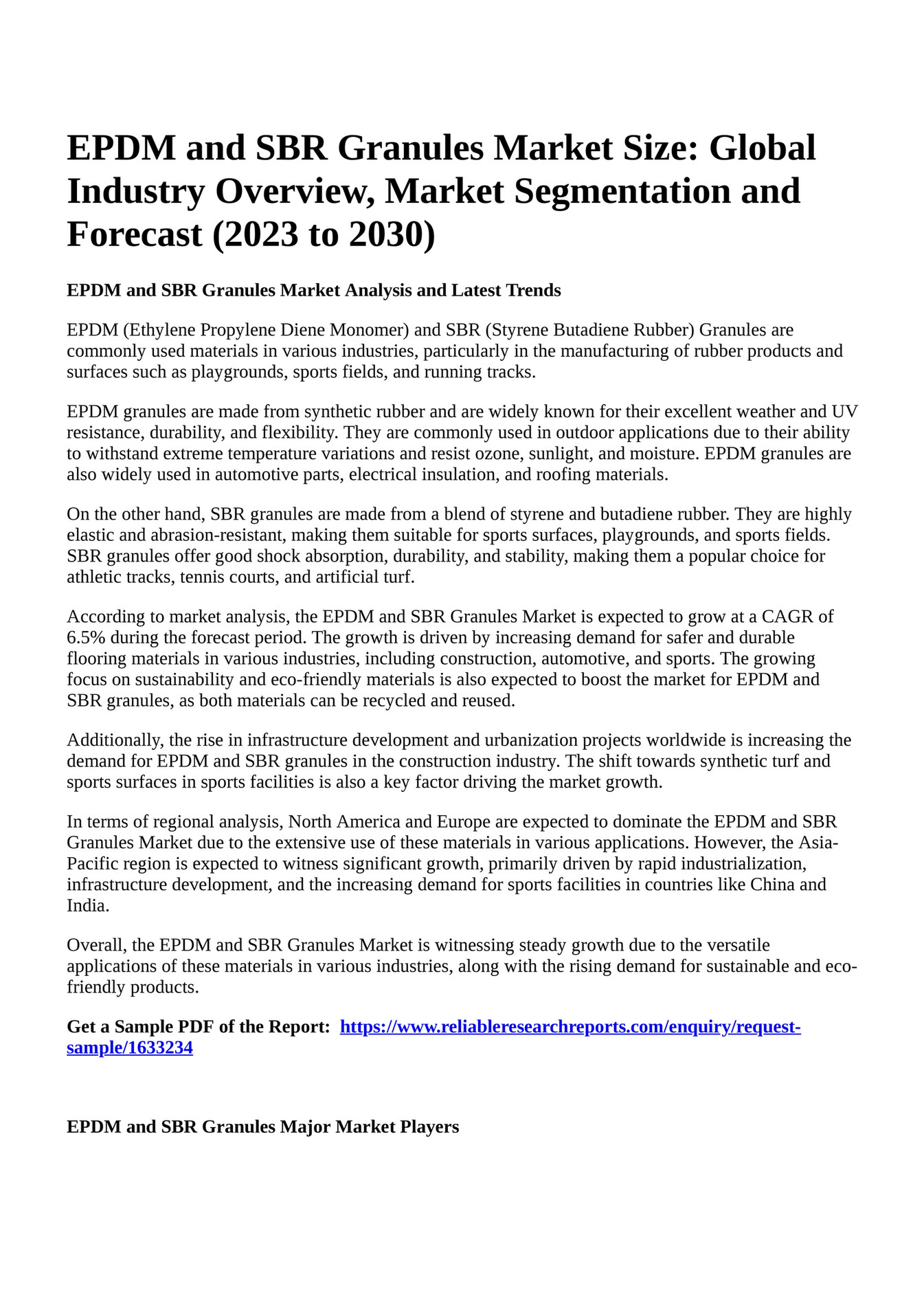The image captures a detailed textual report against a white background. At the top, the prominent and bold heading reads: "EPDM and SBR Granules Market Size, Global Industry Overview, Market Segmentation and Forecast, 2023-2030." Below the main title, there is an additional subtitle in bold that states: "EPDM and SBR Granules Market Analysis and Latest Trends."

The body of the text is divided into seven paragraphs and provides an in-depth analysis of EPDM (ethylene propylene diene monomer) and SBR (styrene butadiene rubber) granules. These granules are widely used in various industries such as construction, automotive, and sports for their impressive properties. EPDM granules are known for their weather and UV resistance, durability, and flexibility, making them ideal for outdoor applications like playgrounds, sports fields, and roofing materials. SBR granules are recognized for their elasticity and abrasion resistance, suitable for sports surfaces and playgrounds due to their shock absorption and stability.

The detailed analysis forecasts a growth rate of 6.5% in the EPDM and SBR granules market from 2023 to 2030, driven by the increasing demand for durable and eco-friendly materials. The report highlights the market's growth potential in North America and Europe, with significant expansion expected in the Asia-Pacific region due to rapid industrialization and development projects.

At the bottom of the page, in bold text, it reads: "Get a Sample of the Report," followed by a blue, underlined hyperlink. This is accompanied by additional smaller black text mentioning "EPDM and SBR Granules Major Market Players."

Overall, the image is a comprehensive textual report providing detailed insights into market trends, segmentation, and forecasts for EPDM and SBR granules, emphasizing their applications and expected industry growth.